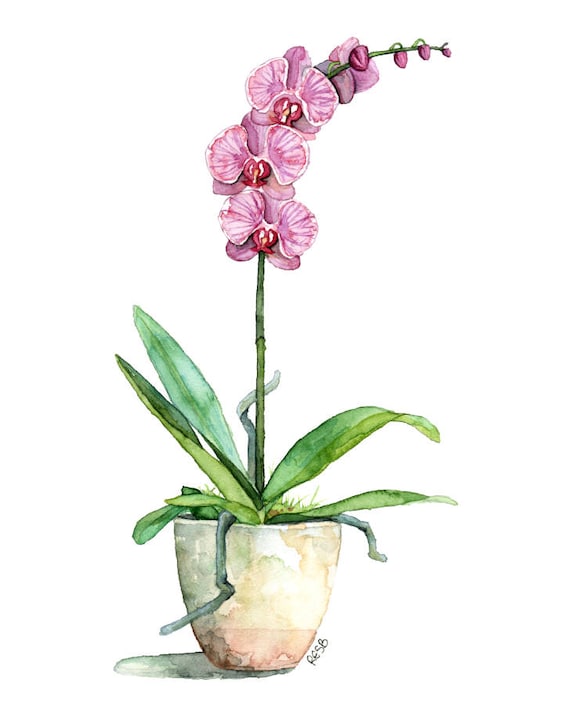This detailed watercolor painting showcases a beautiful orchid in a rounded pot. The orchid features three fully bloomed pink flowers with red stamens at their centers, positioned toward the upper right of the image. There are also four buds that have yet to open and a single blossom seen from the back. The long, graceful stem curves upward and to the right, while six broad green leaves, varying in shades, protrude from the base of the plant, framing it attractively. The rounded pot has a tapered design, wider at the top and narrowing at the base, adorned with beige and light brown hues, including a copper strip near the bottom. Visible roots extend from the pot, adding an extra touch of realism. To the left of the pot, a soft shadow is cast, enhancing the depth of the composition. Near the pot, the text "R-E-S-B" appears, which likely represents the artist's initials. This elegant setting is captured on a white background, emphasizing the delicate and refined nature of the watercolor technique.